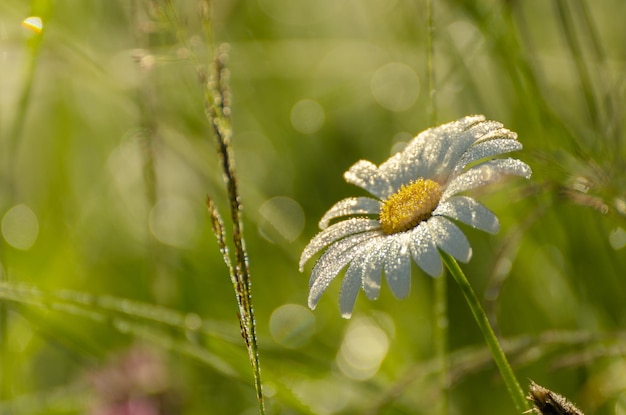The image showcases a close-up view of a white daisy, distinct with its long, slender petals gracefully curving downward and a vibrant yellow center adorned with tiny, feeler-like structures. The daisy stands prominently on a single, green stalk. Surrounding the main flower, the background is artistically blurred, featuring soft hues of green and white intermingled with occasional brown stalks of grass and faint reflections forming circular patterns. A solitary, slightly blurry twig of grass adorned with delicate dewdrops runs adjacent to the daisy's petals, adding a touch of morning freshness to the scene. The blurred backdrop may hint at other elements, like patches of green grasses, potential pinkish-purple flowers, and tree bark textures, but they remain indistinct, enhancing the focus on the daisy.